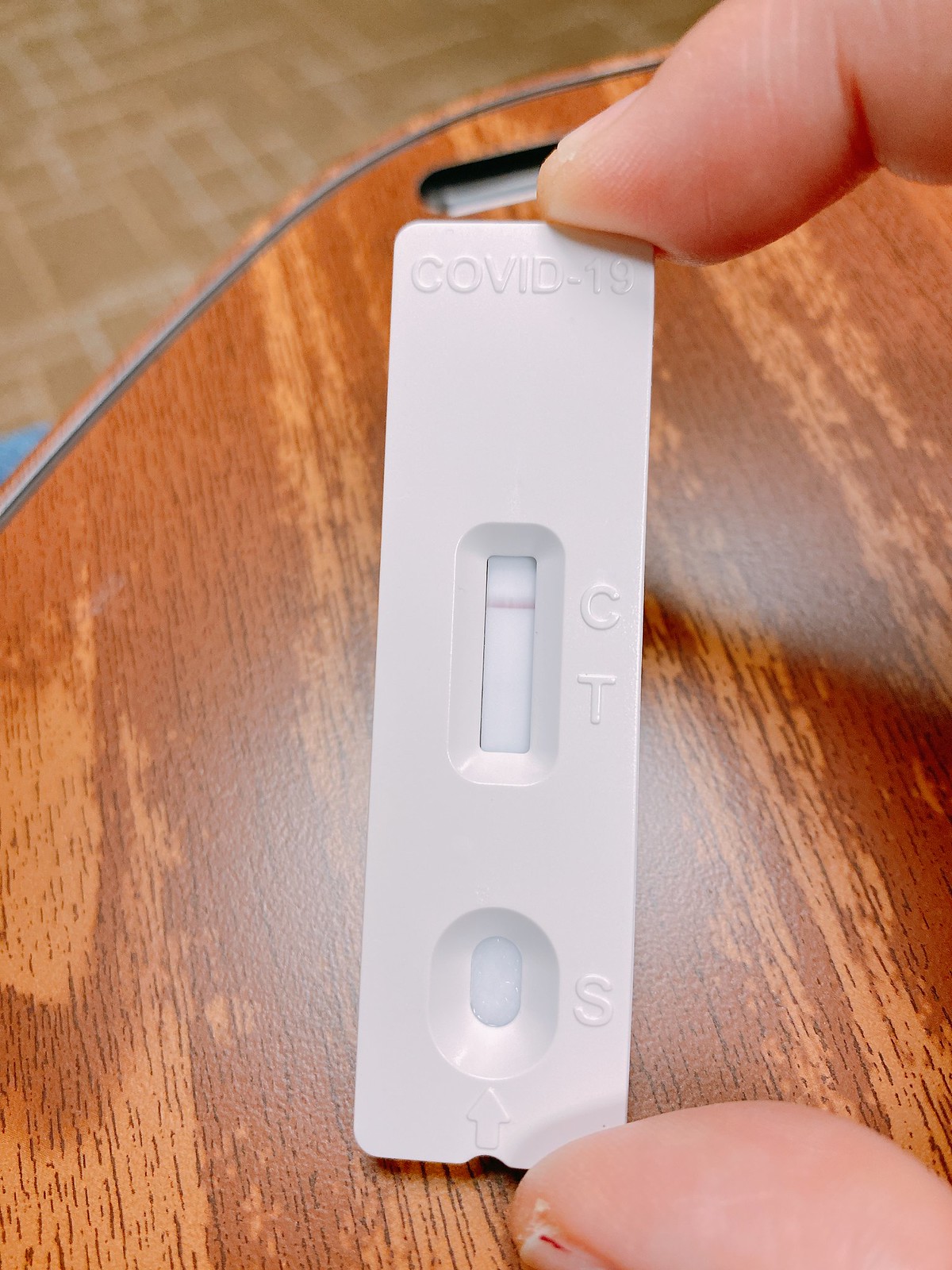The image is a close-up shot showcasing a COVID-19 test strip prominently positioned at the center. The test strip, a vertical white rectangle with a small notch at the bottom center, is held by a thumb and index finger at the bottom right corner. The top of the strip features raised white lettering that reads "COVID-19." Centrally, there is a recessed rectangle with a white background, marked by a faint horizontal red line near its top. Beneath this line is a depressed oval, also white in color. 

The upper left-hand corner of the image reveals a brown and tan carpet with geometric square patterns. The backdrop for the test strip is an orange wooden surface, accented by a silver strip emanating from the left side of the photograph. At the top of the strip, an oblong hole is visible, flanked by lighter orange lines that resemble the wood's grain.